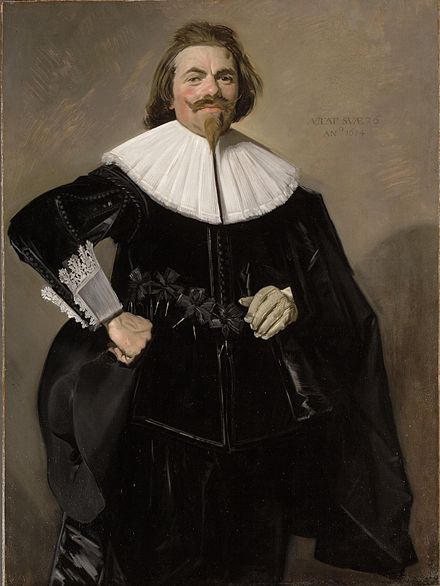The painting entitled "Portrait of Tielemann-Rusterman" by Franz Hals depicts a Baroque style, Dutch Golden Age oil portrait of a Caucasian man standing and gazing directly at the viewer. The subject dons an intricate ensemble of black velvet, featuring a decorative belt with an X pattern, accented by a large, fan-shaped white collar that extends radially from his neck down to his chest and shoulders. His right hand, adorned with a white lace cuff, rests confidently on his hip, while his left, emerging from a black cape draped over his left shoulder, perches on his waist. He holds a black hat in his bare right hand, while his left hand wears a whitish glove. The man's distinguished appearance is further characterized by long, brown, slightly poofy hair brushed back, a mustache turned up at the corners, and a pointed goatee. His face displays a touch of rosiness in his cheeks. The background is an abstract composition of tan and brown brushstrokes, resembling a stucco wall, providing a muted contrast to the detailed and formal attire of the subject. The portrait captures the essence of the era with its meticulous attention to both dress and demeanor.